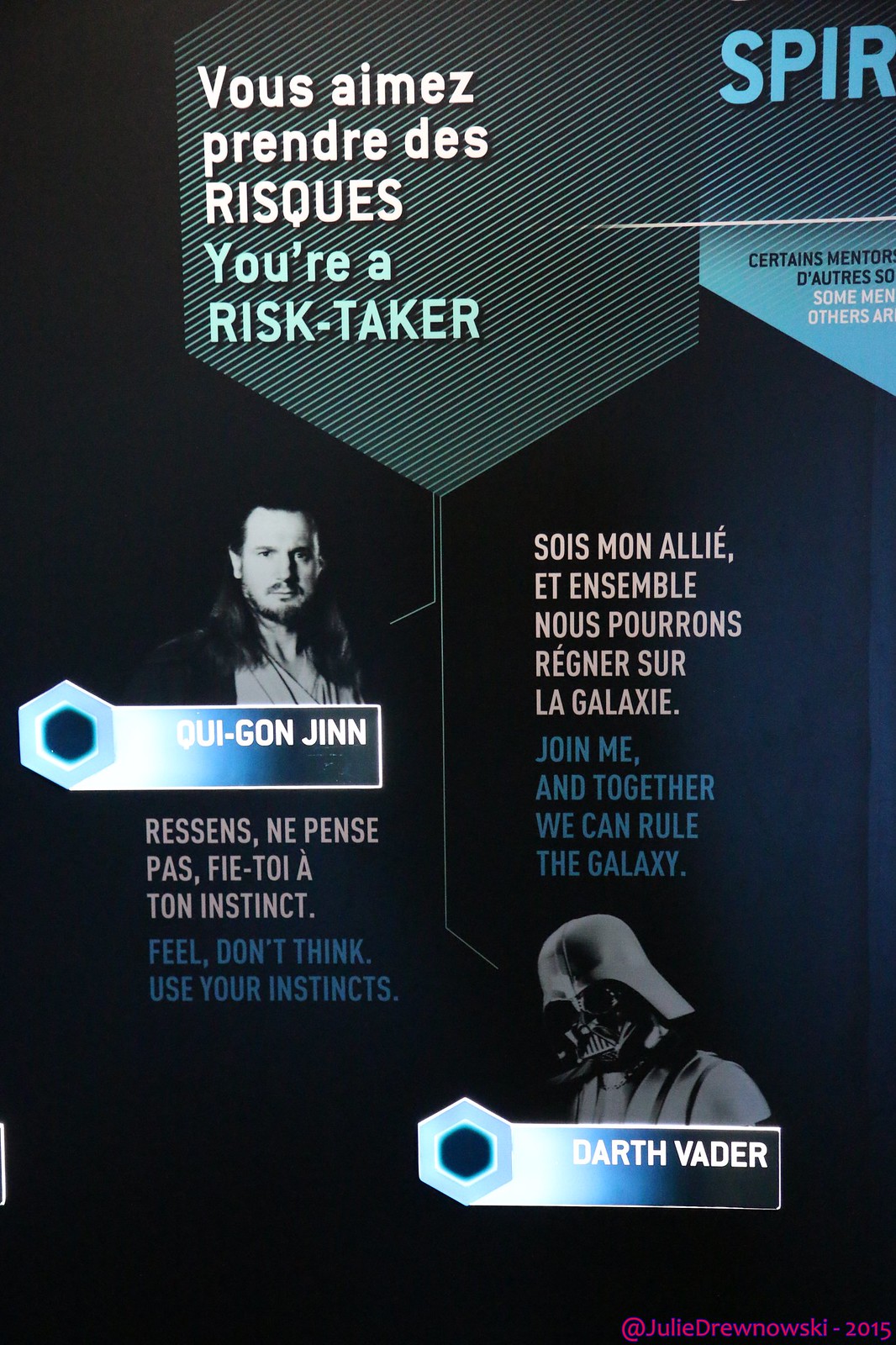The image is a predominantly dark blue, stylized poster with a thematic focus on Star Wars. A light green striped background contrasts with the dark blue at the top. The French text "Vous aimez prendre des risques" translates to "You're a risk-taker" in English. A hexagon pattern also appears in the green lines near the top center, containing fragmented French phrases.

On the right-hand side, a line extends from the middle of the upper announcement down to an image of Darth Vader. Below Vader, in both French and English, it reads: "Join me and together we can rule the galaxy." 

The left side of the poster features a black-and-white image of Qui-Gon Jinn, a character with long, flowing hair looking directly at the viewer. Below his image, within a blue box, his name is spelled out: "O-U-I-Q-U-I-G-O-N J-I-N-N." Further text in both French and English advises: “Feel, don’t think, use your instincts.”

The top right corner of the poster appears obscured but includes part of the text "SPIR." At the bottom of the poster, printed in small red text, is the attribution: "@Julie Drewnowski 2015." The overall appearance of the poster, combined with the iconic Star Wars characters and quotes, suggests that it is promoting a themed event or product related to Star Wars, though the exact nature of the promotion is not entirely clear.